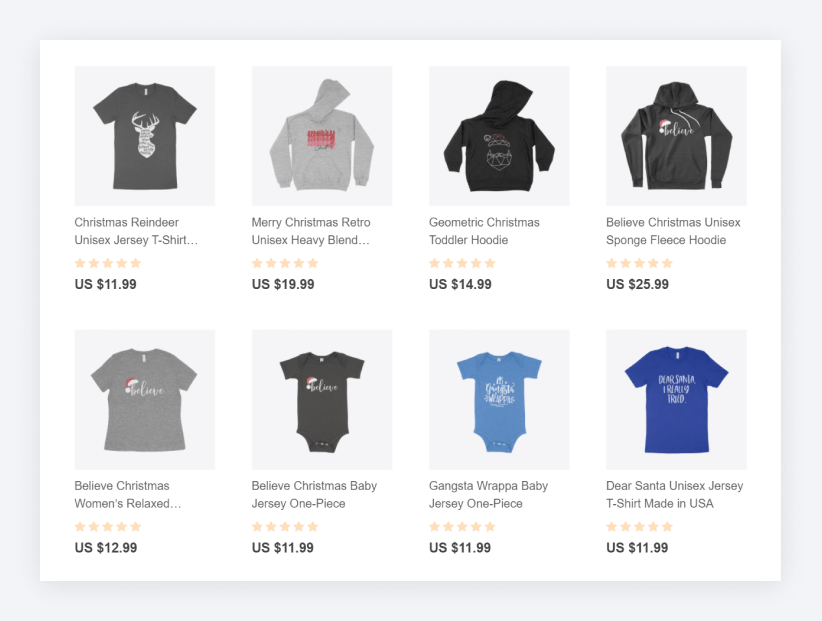The image frame is horizontally rectangular, bordered by a light gray edge. Within this frame, a white, horizontally rectangular box showcases two rows of clothing item listings, with four items per row. Each listing includes a picture of the shirt or garment accompanied by descriptions and prices.

In the top left corner, there's an image and listing for a "Christmas Reindeer Unisex Jersey T-Shirt" priced at $11.99. Next to it is a "Merry Christmas Retro Unisex Heavy Blend Hoodie," available for $19.99. The adjacent listing features a "Geometric Christmas Toddler Hoodie" costing $14.99. Completing the top row is a "Believe Christmas Unisex Sponge Fleece Hoodie" priced at $25.99.

The bottom row starts with a "Believe Christmas Women's Relaxed T-Shirt," available for $12.99, followed by a "Believe Christmas Baby Jersey One-Piece" at $11.99. The next listing is a "Gangsta Wrapper Baby Jersey One-Piece" for $11.99. Lastly, there's a "Dear Santa Unisex Jersey T-Shirt, Made in USA," priced at $11.99.